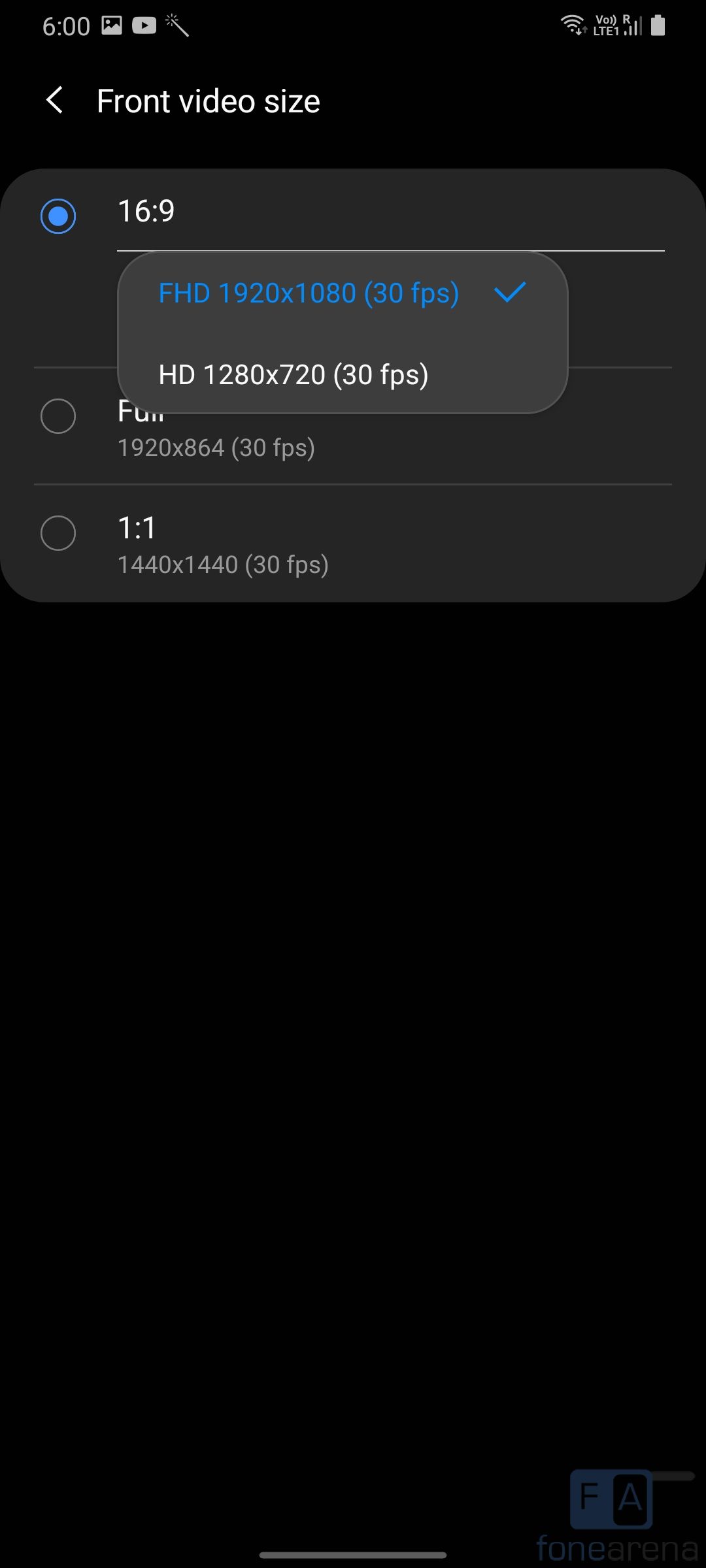Screenshot of a smartphone interface with a black background, captured at 6:00 with a full battery and 3 out of 4 signal bars. The image contains white text that reads "< Front Video Sides" followed by a gray box labeled "16:9" with a selected circle beside it, indicated by a blue fill in the center. Below the "16:9" box, there is a light gray line partially obscured by a pop-up box of a lighter gray color. This pop-up box contains several video resolution options in blue and white text: "FHD 1920x1080 (30fps)" with a blue checkmark, "HD 1280x720 (30fps)", "1920x864 (30fps)", and a circle labeled "111480x1480".